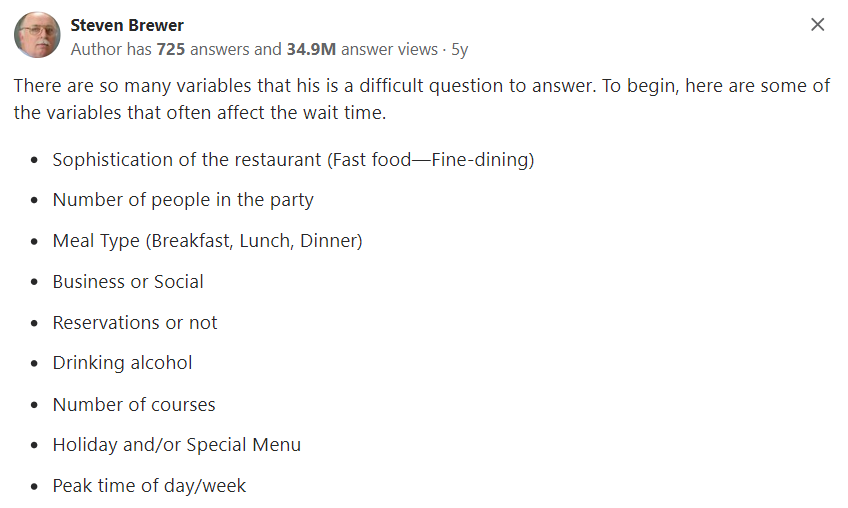A user profile snapshot displays a white screen featuring predominantly grey text. In the top left corner, there's a profile photo of Stephen Brewer, an older gentleman with glasses, a receding hairline complemented by grey hair on the sides, and a white moustache. The profile highlights Brewer's extensive involvement on the platform, noting he has authored 725 answers garnering 34.9 million views over five years.

Below the profile summary, a significant sentence reads: "There are so many variables that this is a difficult question to answer. To begin, here are some of the variables that often affect the wait time." This is followed by a bulleted list detailing factors influencing wait time:

- Sophistication of the restaurant (e.g., fast food vs. fine dining)
- Number of people in the party
- Meal type (e.g., breakfast, lunch, dinner, business, or social)
- Reservations or not
- Drinking alcohol 

This detailed breakdown provides an insightful analysis into the complexities of dining wait times.